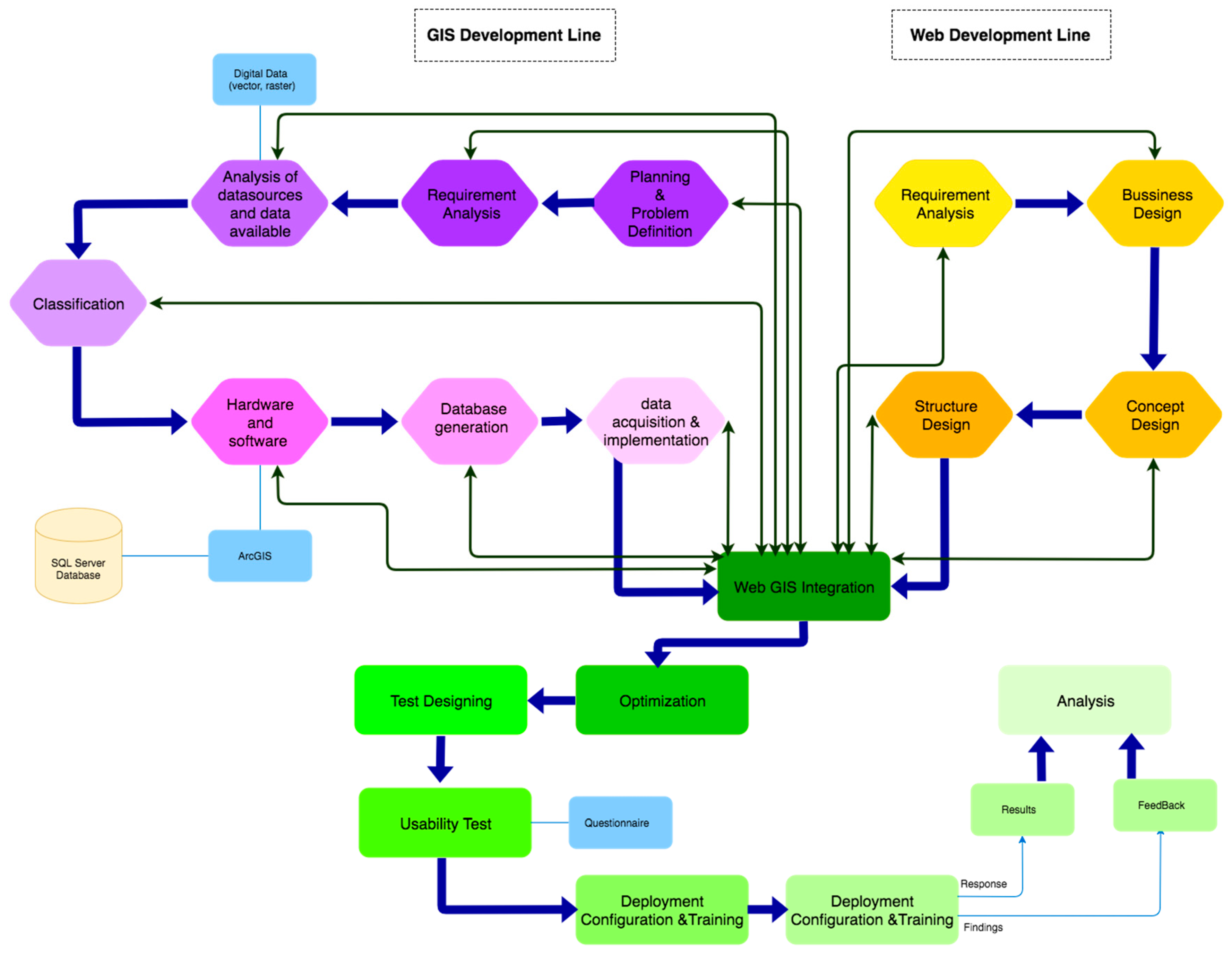The image is a detailed, color-coded flowchart that systematically lays out the processes involved in GIS development and web development. The diagram is predominantly white, and it features two main headers at the top: "GIS Development Line" on the left, outlined in a rectangular dotted line, and "Web Development Line" on the right, similarly bordered. The GIS development section contains various stages such as digital data, vector, raster, analysis of data sources, data availability, requirement analysis, planning, problem definition, data acquisition, implementation, database generation, hardware and software, and classification. 

The web development section includes stages like test designing, optimization, usability tests, questionnaires, deployment, configuration, training, analysis, results, and feedback. In the center of the flowchart, a key integration point labeled "Web GIS Integration" bridges the two development lines and directs the flow downward. 

Color coding enhances the diagram’s clarity: the upper left section is shaded in purple to lilac tones, the upper right in yellow to orange hues, and the bottom part in various shades of green, ranging from forest green to mint green. There are additional elements such as a blue shape that extends from the hardware and software section to a cylindrical SQL server database. 

The flowchart uses thin black arrows to indicate various connections and processes, while thicker blue arrows represent the primary intended pathways through the stages.